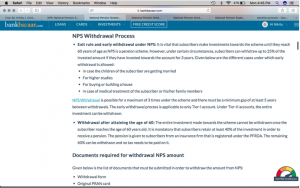This image is a screenshot of a webpage detailing the NPS withdrawal process. At the top, the heading "NPS Withdrawal Process" is prominently displayed. Below this, there are several paragraphs providing information on the process. The words "Edit Rule" are visible, and underneath the "P" and "T" sections, there are multiple bullet points. There is one main bullet point followed by four sub-bullet points. Further down the page, a section of blue text is visible beside more black text.

Continuing downward, there's a single bullet point that introduces an entire paragraph of information. As you move further down, the title "Documents Required for Withdrawal" is displayed, followed by the section "NPS Answer," which has two additional bullet points beneath it. In the lower right-hand corner of the image, there is a multi-colored meter ranging from red to orange, yellow, and green. A black marker on the meter points towards the green section, indicating a favorable status related to the information displayed on the webpage.